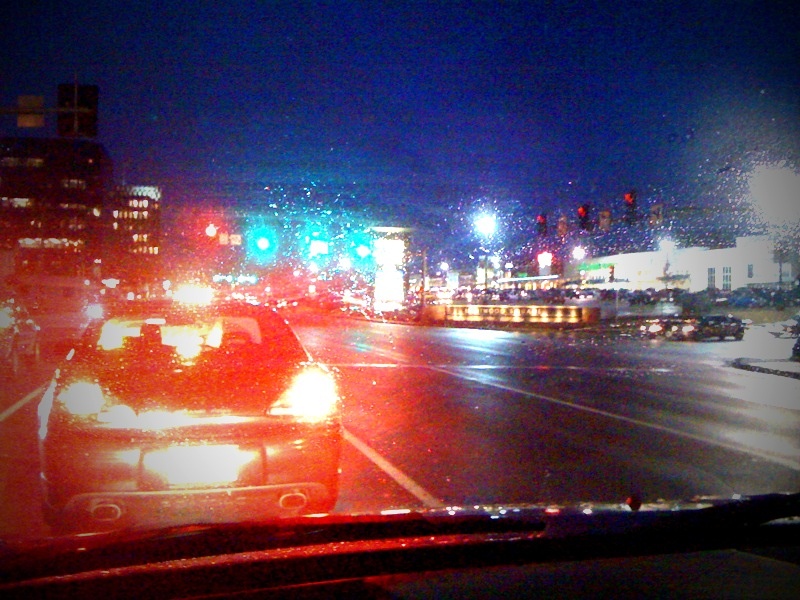This photograph, taken through a car's dashboard-mounted camera, captures a rainy night drive through a city. The car is positioned on the right side of a multi-lane highway with a dark, blue-tinted sky overhead. The windshield, dotted with raindrops, creates a hazy effect, causing the lights to glare significantly. Directly ahead, a smaller sedan is visible, its red taillights glowing intensely and casting a reddish-orange tint over the scene.

In the distance, high-rise buildings lit up with numerous windows form the urban skyline. The wet road reflects various lights, enhancing the overall glow. Multiple traffic lights are seen, primarily red, including a prominent stoplight and a set for the cross street. There's also a billboard near the traffic lights and a white building on the left that might be a car dealership. Overall, the scene has an almost painterly quality, reminiscent of a Leonardo da Vinci painting, blending the urban elements with the dreamy visual effects caused by the rain and reflective surfaces.